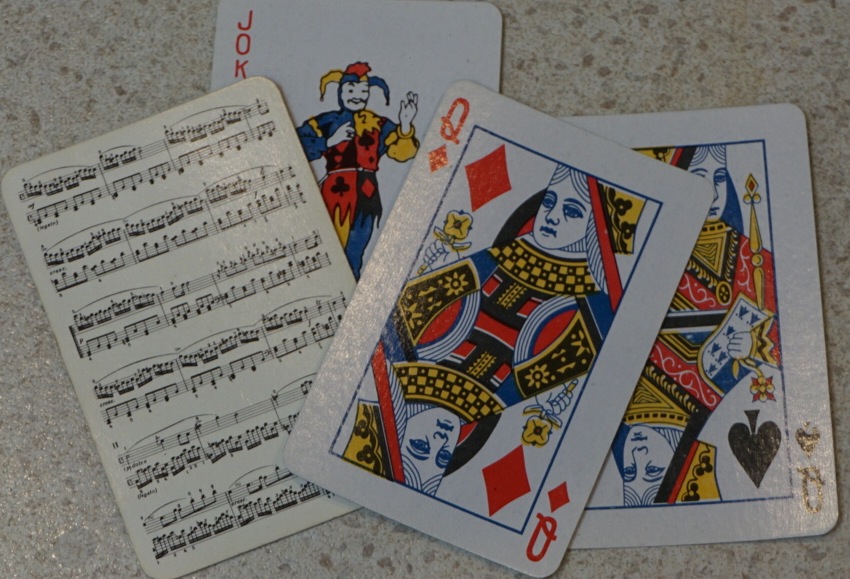A photograph in landscape orientation captures four playing cards lying face up on a light-colored counter decorated with subtle beige and gray flecks. The dim lighting casts soft shadows, creating a cozy ambiance. At the center, the Queen of Diamonds is positioned slightly tilted to the right, overlapping the Queen of Spades on its right. Behind the Queen of Diamonds, on the left side of the image, is a Joker card with its playful design. Partially obscuring the Joker, another unique card is tilted slightly to the left; instead of traditional suits, it features six pairs of staves with musical notes, printed in black on a white background, suggesting it might be a piano score. An overhead light source causes a gentle glare on the Queen of Diamonds, adding a touch of brightness to the otherwise softly lit scene. The viewer’s perspective is from above, offering a clear view of the cards lying flat on the neutral-toned counter.